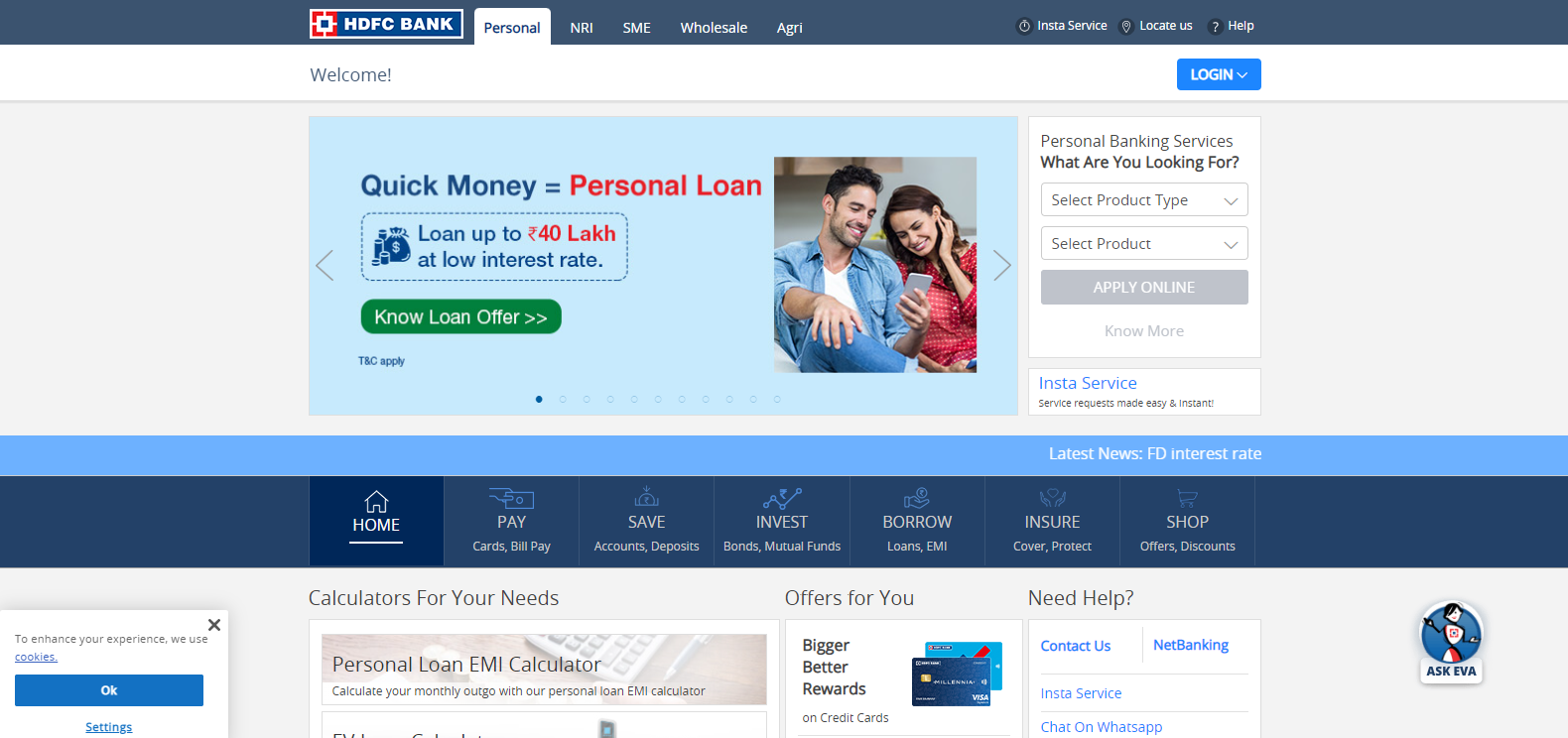Here is a detailed descriptive caption for the provided image:

"The image showcases the homepage of the HDFC Bank website, characterized by a clean and structured layout. At the top, there is a gray header with a white-bordered box set against a blue background that prominently displays the HDFC Bank logo, featuring a distinctive red, white, and blue pinpoint design. This header also includes navigation options such as 'Personal,' 'NRI,' 'SME,' 'Wholesale,' and 'Agri,' along with shortcut links for 'Insta Service,' 'Locate Us,' and a 'Help' button on the right.

Just below the header, the website greets visitors with a 'Welcome' message and a blue 'Login' button. The central portion of the image comprises a blue background section highlighting a promotional message: 'Quick Money = Personal Loan. Loan up to 40 LAKH at a low interest rate.' This is accompanied by options for users to select product types and apply online, with 'Apply Online' and 'Know More' buttons available.

Additionally, there is a highlighted blue banner announcing 'Latest News: FD Interest Rate.' Beneath this banner, there are clickable categories such as 'Home,' 'Pay,' 'Save,' 'Invest,' 'Borrow,' 'Insure,' and 'Shop.' The website further offers tools like a 'Personal Loan EMI Calculator' and lists enticing offers with the slogan 'Bigger Better Rewards.' For customer assistance, it provides contact details for NetBanking, Insta Service, and a chat option via WhatsApp."